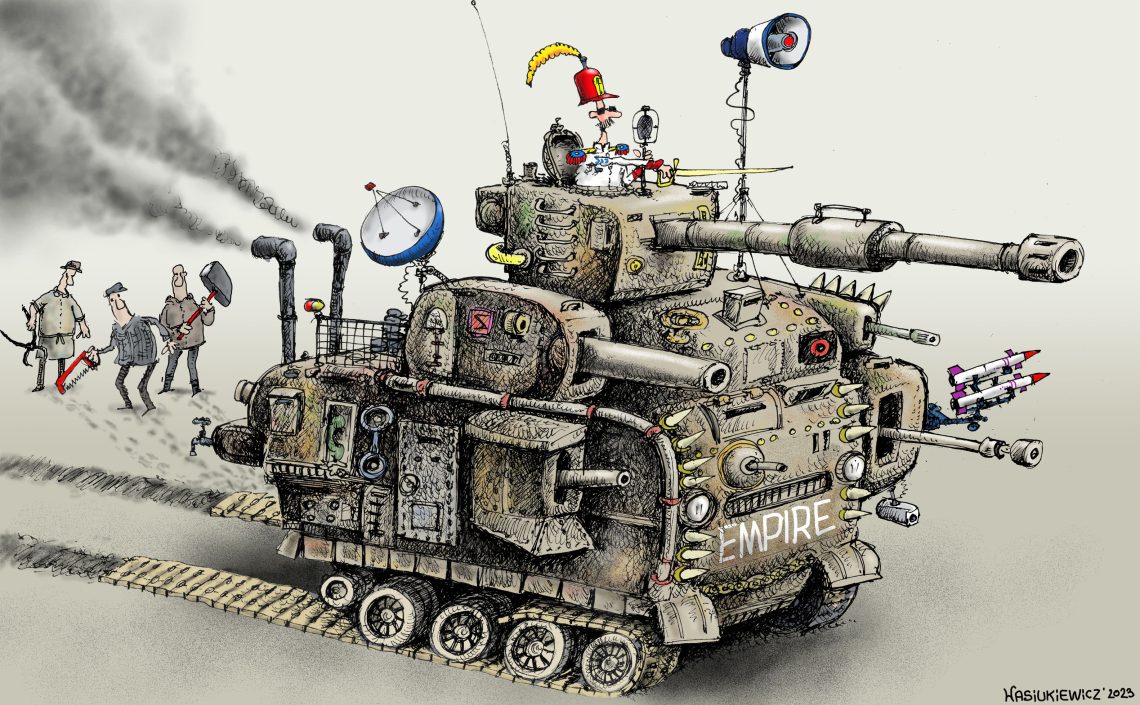The image is a horizontally aligned rectangular political cartoon set against a light gray background, dated 2023, and signed by W-A-S-I-U-K-I-E-W-I-C-Z. Dominating the center of the scene is a large, elaborate tank bearing a vintage design akin to those from the end of World War I and the early stages of World War II, yet heavily modified with a myriad of guns, missiles, and spikes, giving it a dystopian, Mad Max-esque appearance. The tank features a label "EMPIRE" in bold white letters on its front and is equipped with a satellite dish pointing upward.

Atop the tank sits a small, caricatured figure dressed in a white military uniform, adorned with a red hat featuring a prominent yellow feather. The figure, wielding a gold sword pointed forward, has a distinctive long nose, narrow face, and mustache. Surrounding the tank, on the left side, are three men depicted as farmers or workers, each holding a large tool—a hammer, a handsaw, and a wrench—and watching in apparent confusion as the tank proceeds forward with its track dislodging from the wheels. The scene overall conveys a chaotic juxtaposition of advanced military might and simpler, agrarian figures, suggesting a satirical take on power dynamics and overreach.